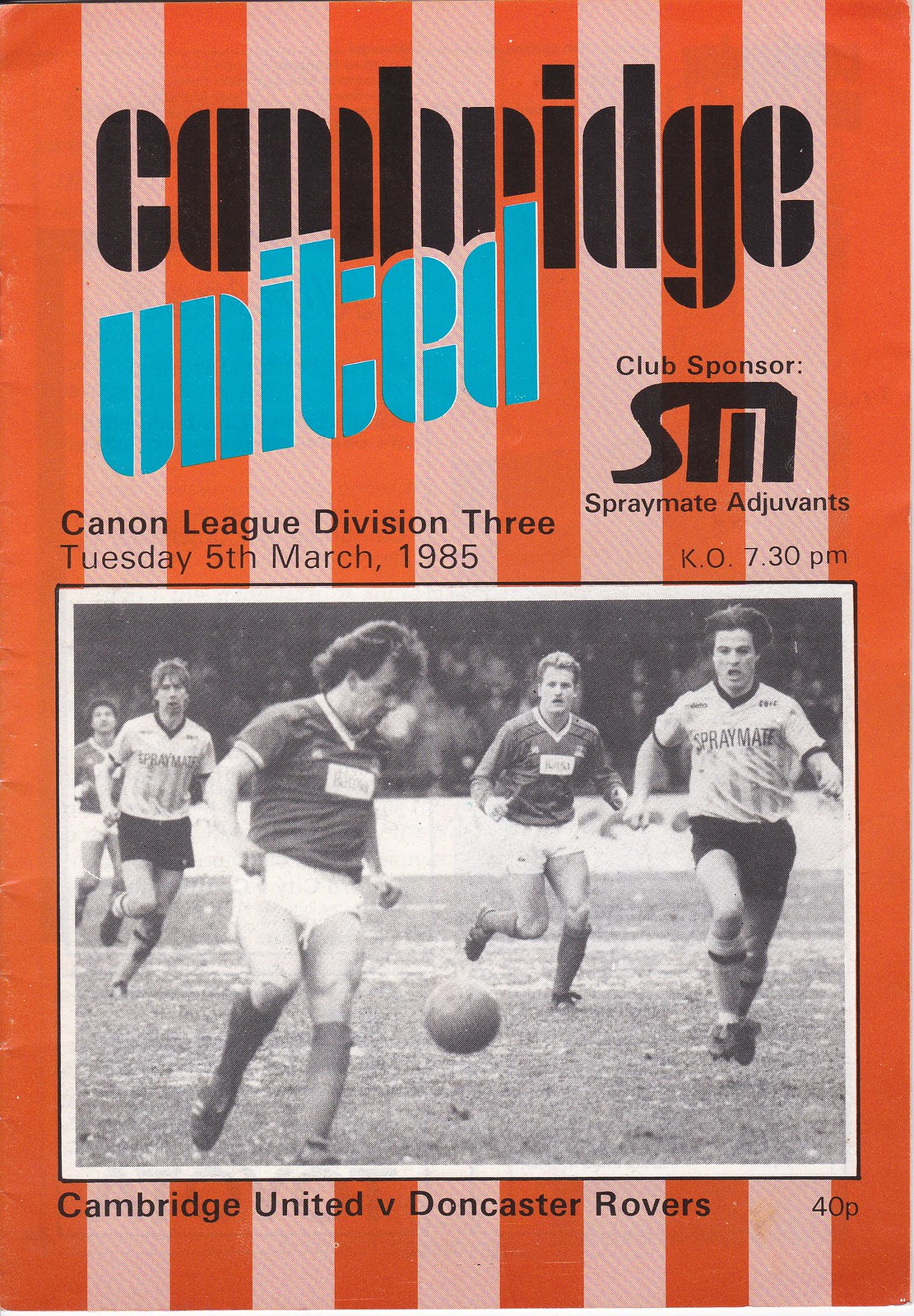This image is the front cover of a Cambridge United football program for a match against Doncaster Rovers in the Canon League Division 3, scheduled for Tuesday, March 5th, 1985, with a kickoff at 7:30 p.m. The cover features vertical stripes of orange and pink in the background. At the top, "Cambridge United" is prominently displayed with 'Cambridge' in black lettering and 'United' in teal blue. Below the club name is the sponsor "Spraymate Adjuvants." The main section includes a black-and-white photo of six soccer players, with one player slightly to the left center, appearing to chase a ball in mid-air. The field is visible at the bottom of the image with grass, and the top shows barriers and spectators in the stands. The setting clearly indicates that this is a program cover, with the details "Cambridge United vs. Doncaster Rovers" and the price "40p" noted below the image. The primary colors used are orange, pink, black, white, and blue.